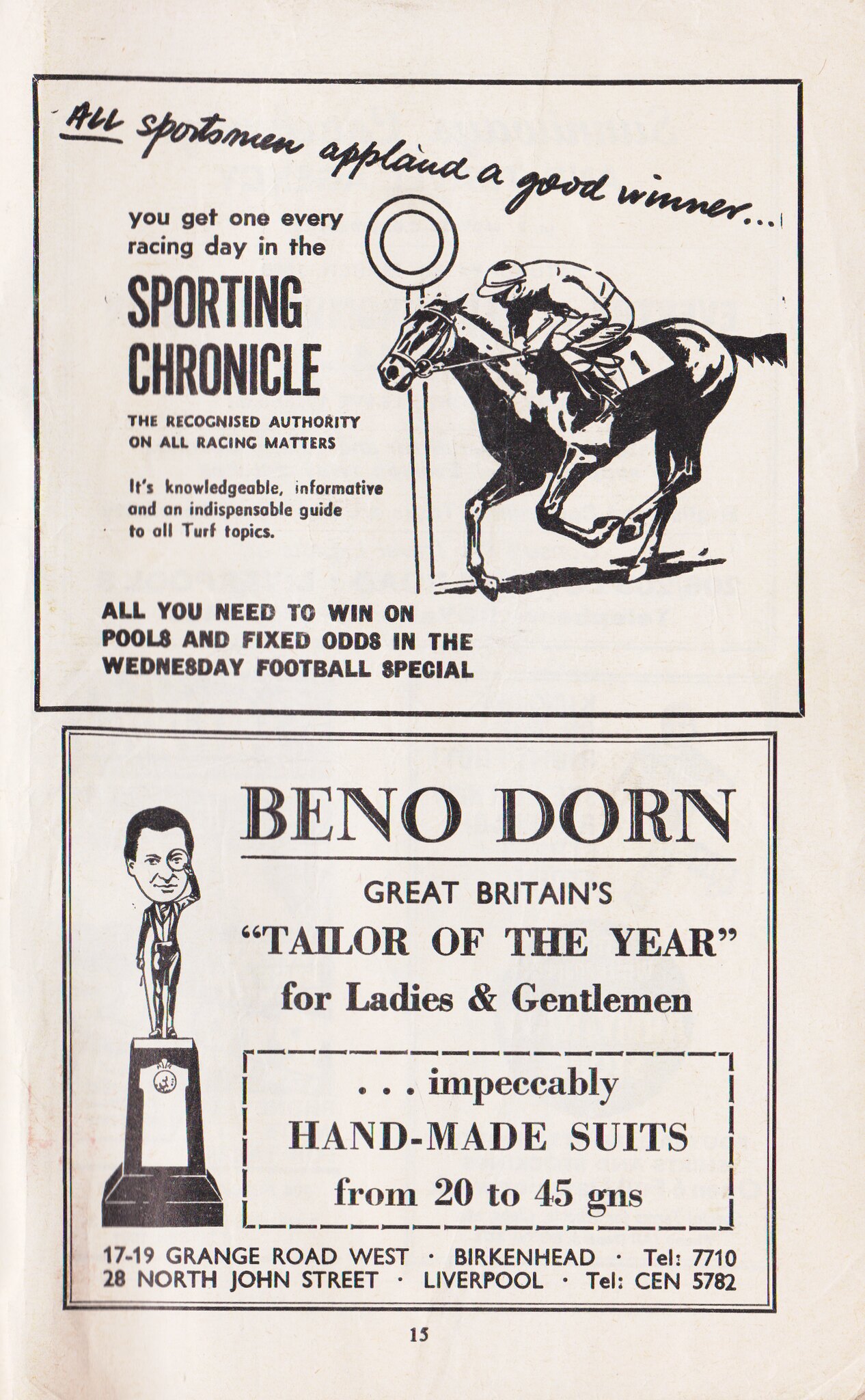In this black and white image of a printed advertisement on a white background, two main sections are bordered by thin black lines. The top section features the bold, cursive heading, "All sportsmen applaud a good winner," with the word "ALL" underlined and capitalized. Directly below this header, on the left, promotional text extols the "Sporting Chronicle" as the ultimate authority on all racing matters, describing it as knowledgeable, informative, and an indispensable guide for turf topics, pools, and fixed odds, especially for the Wednesday football special. On the right side of this section, a black and white drawing depicts a jockey riding a numbered racehorse.

The bottom section of the advertisement shifts focus to fashion, highlighting "Ben O'Dorn, Great Britain's Tailor of the Year for Ladies and Gentlemen." This text is in bold and promotes impeccably handmade suits priced between 20 to 50 GNS. Below this, contact information appears for locations on Grange Road West, Birkenhead, and North John Street, Liverpool. To the left of this text, a drawing, resembling a statuette of a man atop a trophy, adds visual interest to the ad.